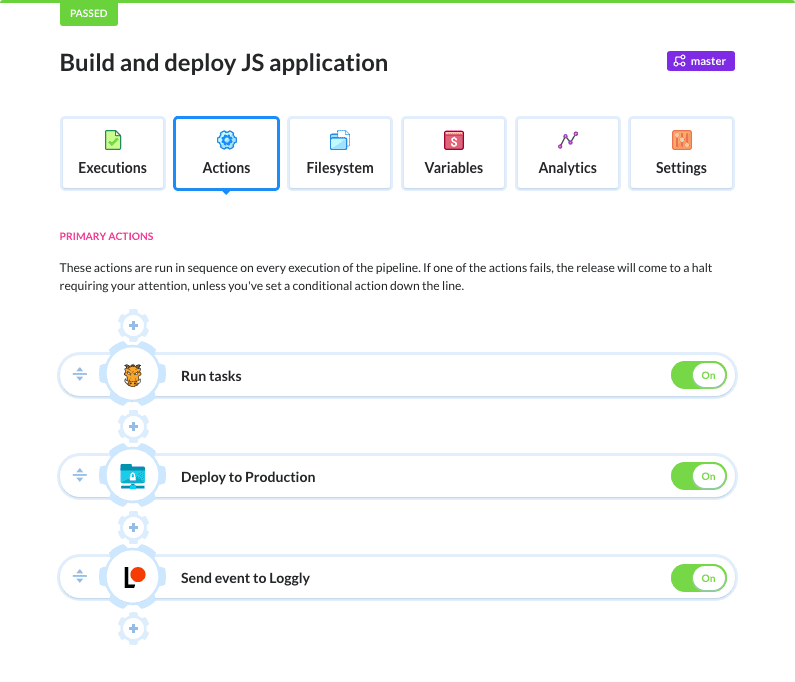The image displays a web application interface with various elements. At the top of the screen, a thin green line stretches across, indicating a successful operation. In the upper left-hand corner, a small green box features white text that reads "PASSED," signifying the successful build and deployment of the JavaScript application.

On the far right, a white three-pronged icon labeled "MASTER" sits atop a purple button. Below these elements, a navigation menu offers several options: Executions, Actions, File System, Variables, Analytics, and Settings. The Actions button is highlighted, indicating that the displayed content pertains to this category.

Under "Primary Actions," the interface explains that these actions are executed in sequence during each pipeline run. If any action fails, the release process is halted until the issue is addressed, unless a conditional action is specified later in the sequence.

The following actions are listed:

1. **Run Tasks:** This action is currently toggled on, with plus and minus buttons to adjust settings.
2. **Deploy to Production:** This action is also activated, featuring plus and minus buttons for configuration.
3. **Send Event to Loggly:** This action is enabled as well.

The comprehensive details help ensure users understand the current state and sequence of actions within the pipeline.